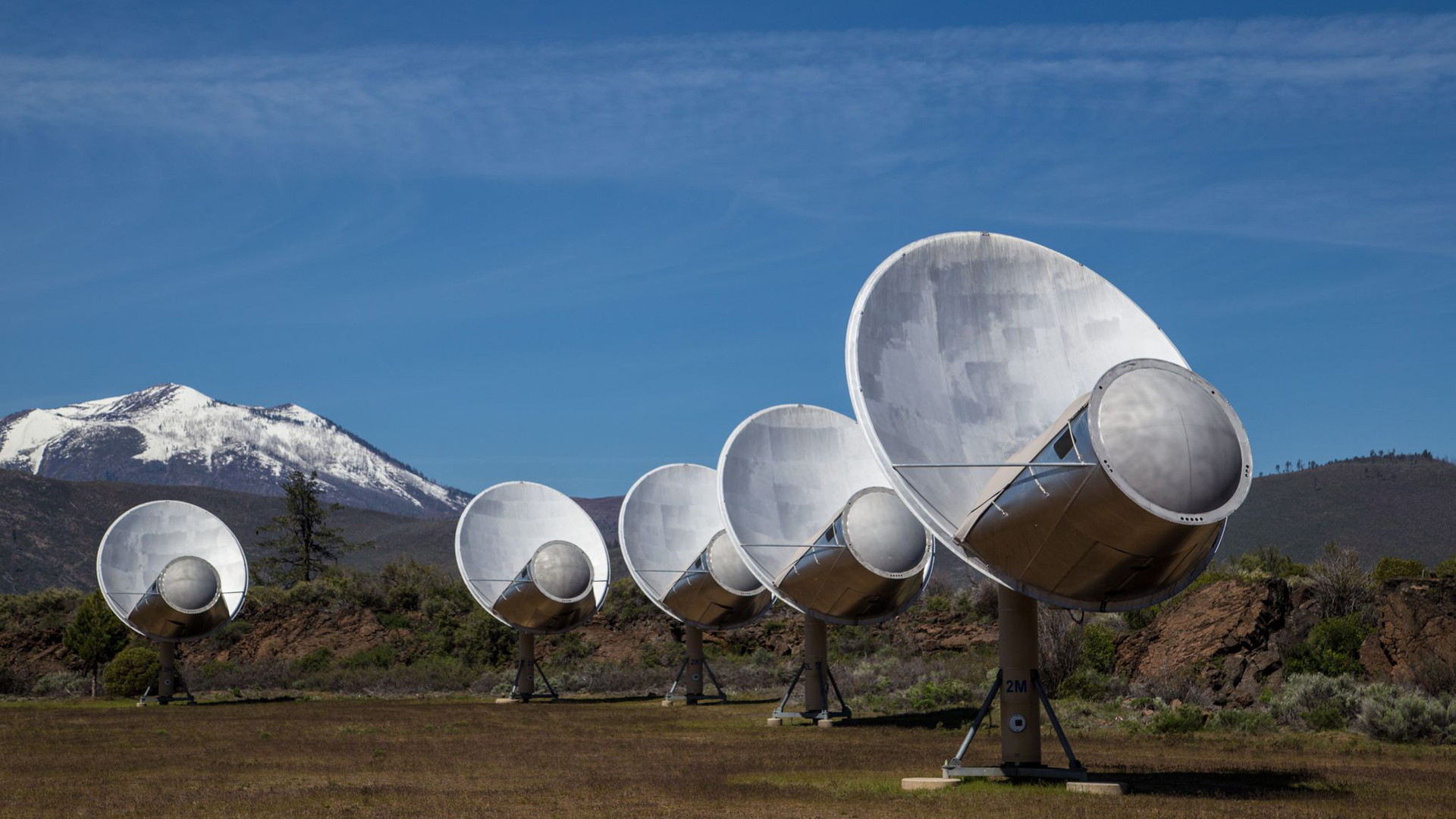This photograph captures a serene countryside scene, possibly in Colorado, featuring a vibrant light blue sky dotted with faint, wispy clouds. Two prominent mountains dominate the background: one on the left is capped with snow covering approximately 75% of its surface, while the other mountain remains lush and green. In the mid-ground, a solitary tree stands beside a rugged, rocky area. Closer to the foreground, five satellite dishes are arrayed in a slightly scattered formation. These satellite dishes, notable for the large barrels protruding from their bases, rest on a flat terrain where the grass appears brown and dead, with sparse green patches peeking through. The overall setting feels isolated, with no buildings or houses in sight, enhancing the sense of tranquility amidst the majestic Colorado mountains.